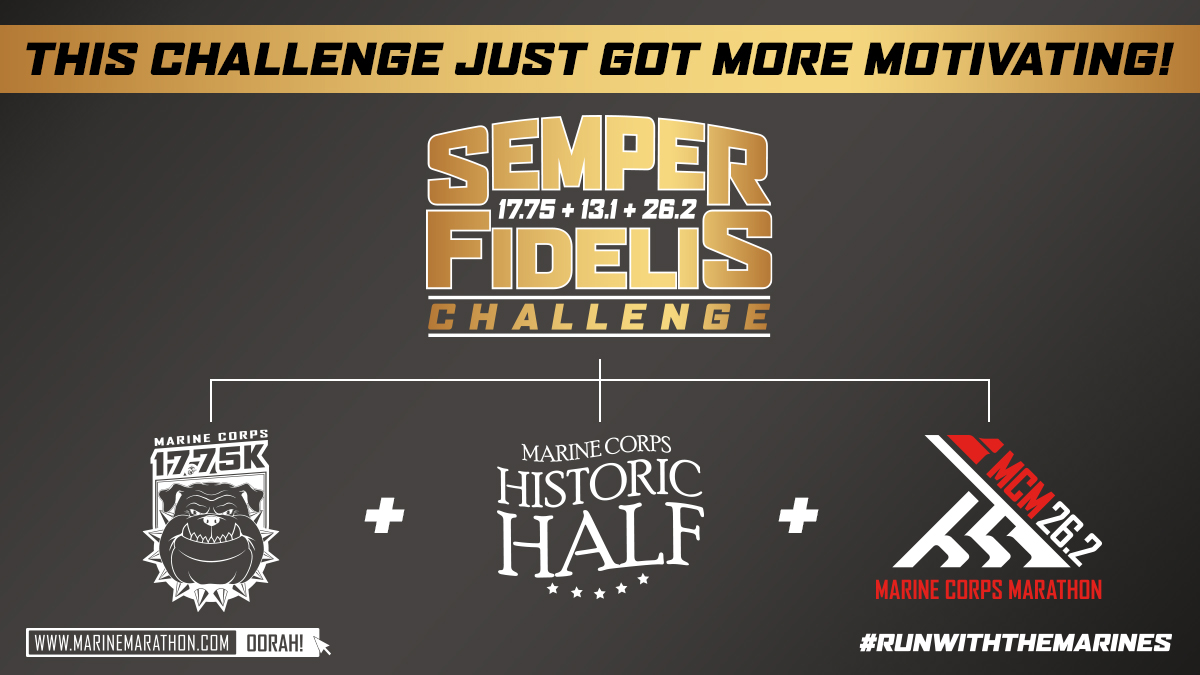The image is a visually striking advertisement for a marathon event organized by the Marine Corps, with a dark gray background. Dominating the top of the poster is a bold motivational phrase in yellow, "This Challenge Just Got More Motivating." Below this phrase, the main title "Semper Fidelis Challenge" is prominently displayed in gold lettering with "Semper" arched above "Fidelis." Between these words are three numerical sequences representing different race distances: 17.75, 13.1, and 26.2.

These numbers correspond to three separate running challenges highlighted in the graphic. The first is the Marine Corps 17.75K, symbolized by a logo featuring a bulldog with a spiked collar. The second is the Marine Corps Historic Half Marathon, represented by five stars arranged in an arch. Finally, the third challenge is the Marine Corps Marathon (MCM), which is a classic 26.2-mile race.

Near the bottom of the poster, additional details include the website address "www.marinemarathon.com" on the left and the hashtag "#RunWithTheMarines" on the right, encouraging participants to join and share their experiences. The overall design uses a combination of gold and white text to create a sense of honor and excitement around participating in these prestigious events with the Marines.